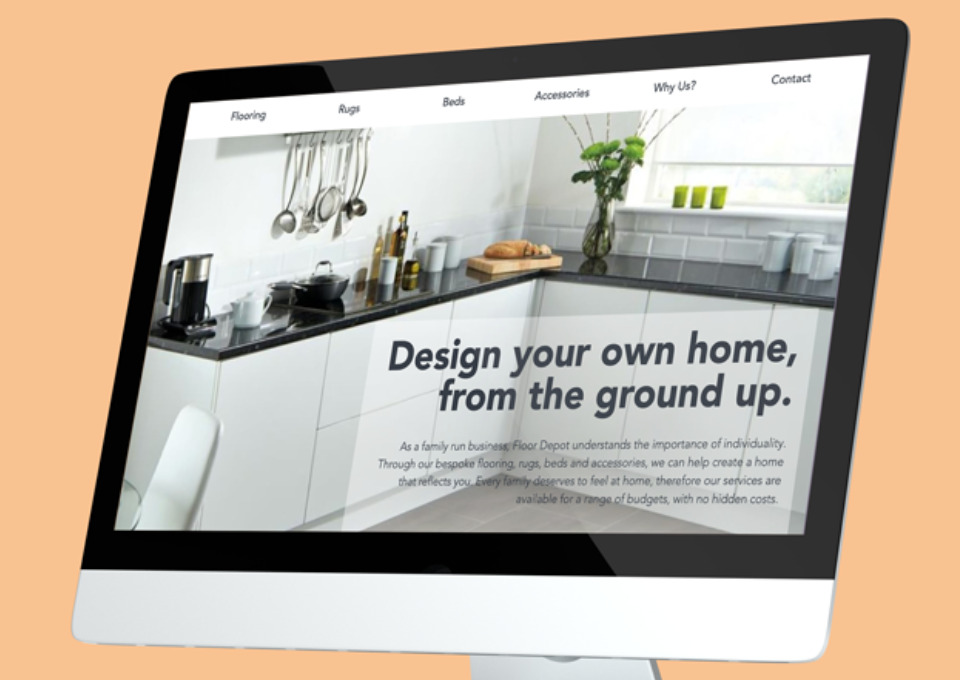The image features a pink-colored background with a tablet or computer monitor prominently displayed. The monitor has a white border along the bottom and a black, rectangular edge around the top and sides. At the top of the screen, there is a navigational bar with clickable options labeled from left to right: Flooring, Rugs, Accessories, Why Us, and Contact.

The scene depicted on the monitor is a kitchen interior. The kitchen has white walls comprised of white bricks on the lower section and a drywall-type material on the upper section. On the right side of the kitchen, there is a window with partially pulled-up blinds, and three cups are placed on the windowsill.

Beneath the window is a black marble countertop adorned with a plant in a vase. The cabinetry consists of white doors and drawers, contributing to the room's clean and modern aesthetic.